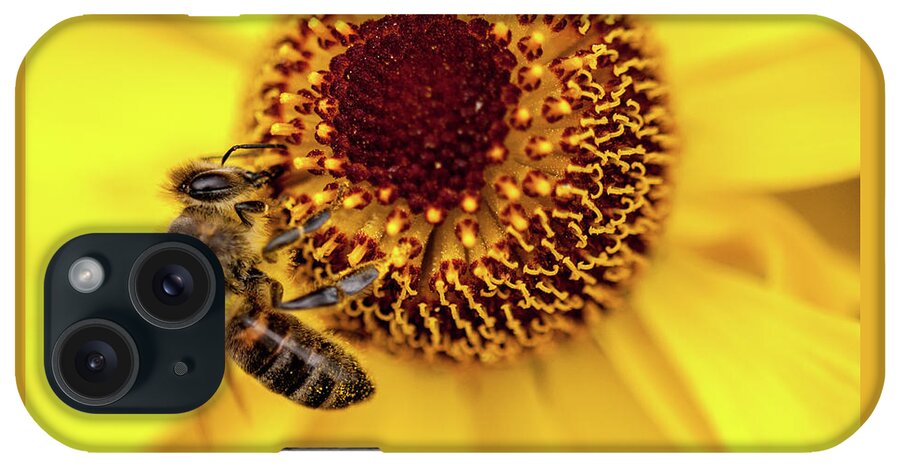This close-up stock photograph depicts the back of a black iPhone, held horizontally to reveal its dual camera setup and flash within a square-like arrangement in the upper left corner. The phone is sheathed in a vibrant phone case dominated by an extreme close-up image of a sunflower's center, showcasing the intricate details of the flower and its visitor. The flower's silky yellow petals surround its dark yellow and reddish fuzzy stamen center. Perched in the middle of the flower is a bee with visible legs, stinger, body, head, and antennae, appearing to feast on the flower. The compelling image captures the textures and colors of both the flower and the bee, highlighting the natural artistry of the scene.